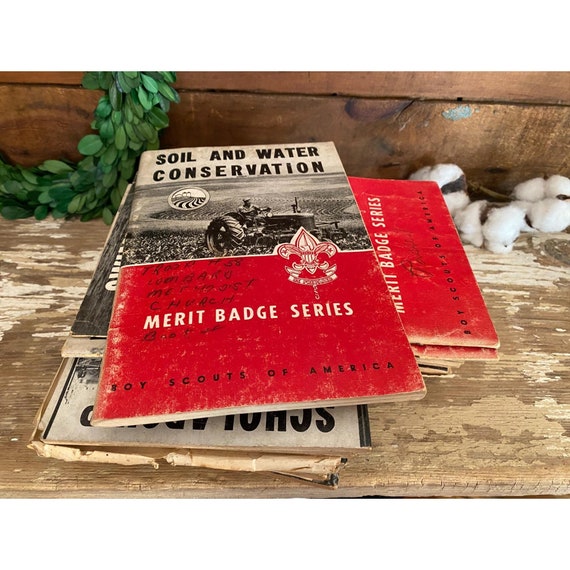The photograph features a weathered stack of small, old paperback pamphlets or books, prominently situated on a weathered, tan-colored wooden table or bench, which appears to be sitting outside. The top book is titled "Soil and Water Conservation" from the Merit Badge Series of the Boy Scouts of America, adorned with the emblem crest on the right side. It features a black-and-white photograph of a man on a tractor. The book's cover is red on the bottom half with white and black text. Surrounding the books is a mix of natural elements, including green leaves to the left side and a backdrop of a brown wooden wall, indicative of the bench's flaking paint and outdoor setting. Further details reveal that there are several other books in the stack, though their titles are indiscernible. The scene evokes a sense of aged study materials amidst a rustic, natural environment.